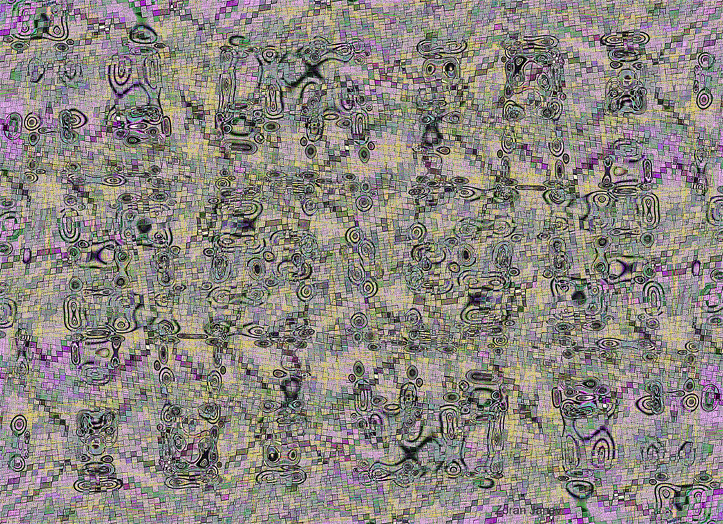This full-color image features an intricate and highly detailed design, characterized by a chaotic yet captivating arrangement of geometric shapes, primarily squares, in various shades of purple, yellow, and black. This seemingly unstructured artwork comprises both tiny and larger imperfect squares, each delineated by fine gray or black lines, creating a mosaic-like pattern. The squares are interspersed with whimsical, swirling black lines—some thick, some thin—adding to the dynamic and unpredictable feeling of the piece.

The background exhibits a purplish and beige hue that complements the squares' diversity, creating an overall busy and vibrant composition. This modern art piece, reminiscent of works found in contemporary art museums, is abstract and not signed by any artist. Upon closer inspection, one might discern faces, animals, or objects within the geometric patterns, hinting at a deeper complexity beneath the apparent chaos. The artwork's spontaneity and multitude of colors ensure that the viewer's eye is constantly drawn from one intriguing detail to the next, making it difficult to focus on any single part for too long.